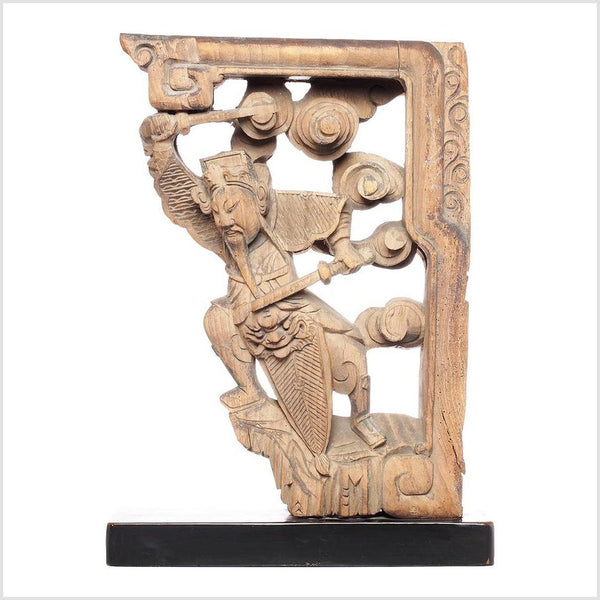This is an intricately carved wooden or stone depiction of a traditional Chinese or Asian warrior. The carving rests on a black rectangular base, which may be metal or wood, lightly trimmed in brown at the edges. The background of the image is pure white, providing a stark contrast to the detailed artwork. The warrior, possibly a samurai due to his traditional armor and headpiece, stands poised on what resembles a cliff edge. His dynamic stance includes one sword held aloft above his head and another pointed forward at his waist. Swirling patterns, potentially symbolizing wind, encircle him, with various holes visible through these swirls and the spaces between his limbs. His armor features prominently, including shoulder guards and a loin piece adorned with a lion's face. He has a long, thin beard and appears connected to the top section of the carving by attachment pieces, suggesting a suspended or framed composition. The overall effect is one of motion and tension, capturing a moment frozen in time, possibly as part of an ornate set of bookends or as a standalone decorative piece.